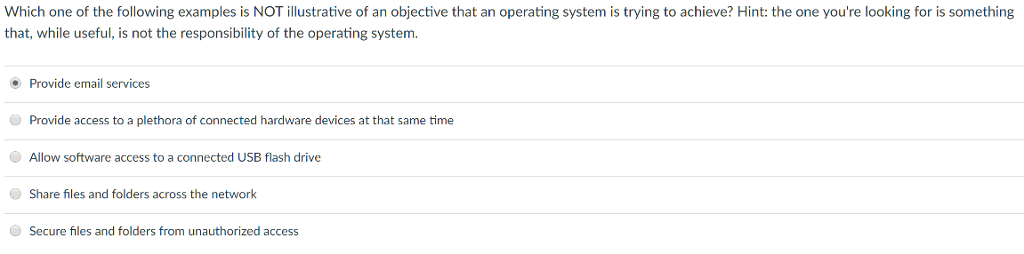This image is a screenshot from a quiz website featuring a specific question displayed to the user. The question asks, "Which one of the following examples is not illustrative of an objective that an operating system is trying to achieve?" A hint is provided, indicating that the correct answer is something useful but not the responsibility of the operating system. Below the question, five options are listed:

1. **Provide email services** (the option selected by the user),
2. Provide access to a plethora of connected hardware devices simultaneously,
3. Allow software access to a connected USB flash drive,
4. Share files and folders across the network,
5. Secure files and folders from unauthorized access.

The user's selection, "Provide email services," is highlighted and aligns with the hint given.